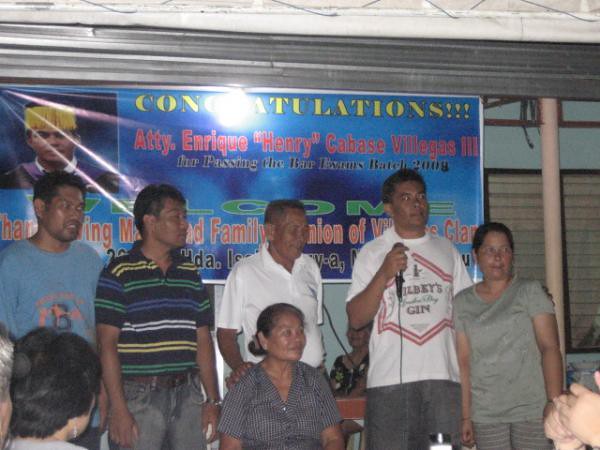A group of five people stand together in front of a celebratory banner, with two additional individuals partially visible in the foreground. Starting from the left, the first person is a man with dark black hair, wearing a blue shirt adorned with a black bee, looking towards the right. Next to him stands a man in a black shirt featuring stripes of yellow, green, blue, and white, along with blue jeans, also facing right. The third in line is an older man with grayish hair at the sides, dressed in a plain white shirt. Beside him is another man in a white shirt marked with an emblem and the word "Jin" at the bottom, holding a microphone. The fifth person is a lady with black hair pulled back, wearing a gray shirt and leaning into the man next to her.

In the foreground on the left, the back of a woman's head with black hair and wearing an earring is visible, while on the right, a pair of hands are seen sticking out into the corner.

The banner behind them has a blue background and reads, "Congratulations Attorney Enrique Henry Cabanse Villegas III for passing the Bar Exam Bar 2009," with a bright white reflection in the word "Congratulations." On the upper left corner of the banner is a picture of Enrique Henry Cabanse Villegas wearing a yellow headband. Additionally, there is a pink post visible on the right side of the image.